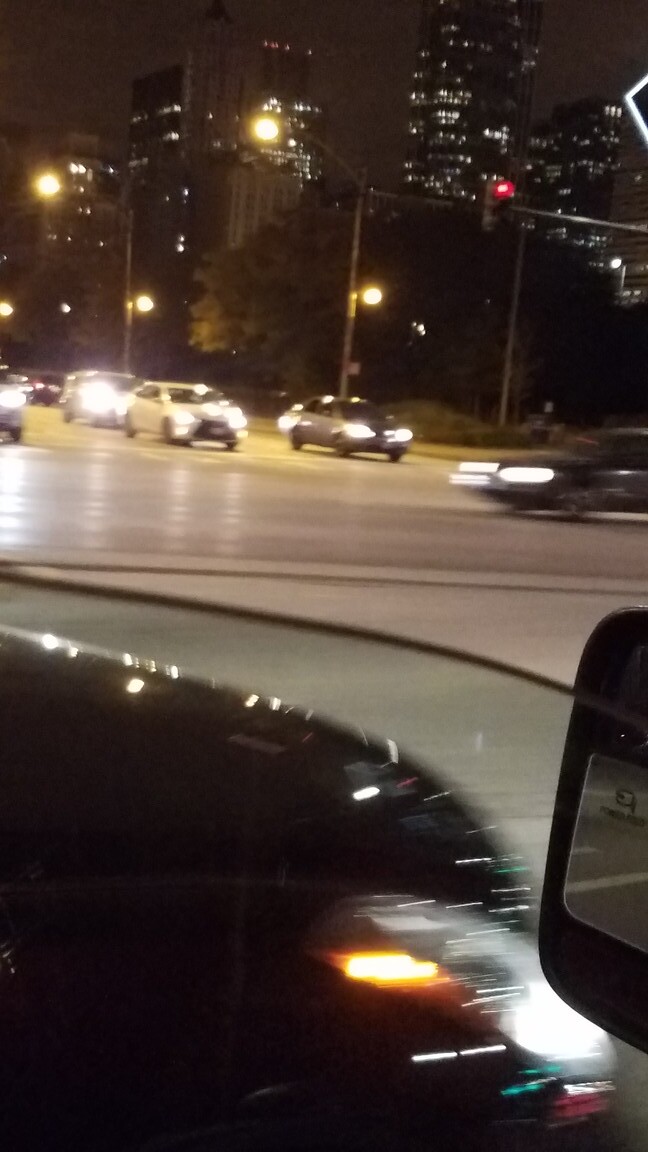The nighttime image appears to be taken from inside a moving car by the passenger, capturing the blurry dashboard with various lights—yellow, white, green, and red. Through the windshield, an intersection scene unfolds. Vehicles, including a black car with its lights on crossing the opposite lane, and several sedans—white, silver, and another unclear car—are queued at a red light. The street is illuminated by four yellowish-white street lights mounted on two silver poles. The sky is dark, adding contrast to the city lights and highlighting the tall buildings adorned with white lights both inside and out, evoking a bustling downtown ambiance. Trees with heavy greenery frame the street, completing the vibrant urban nightscape.